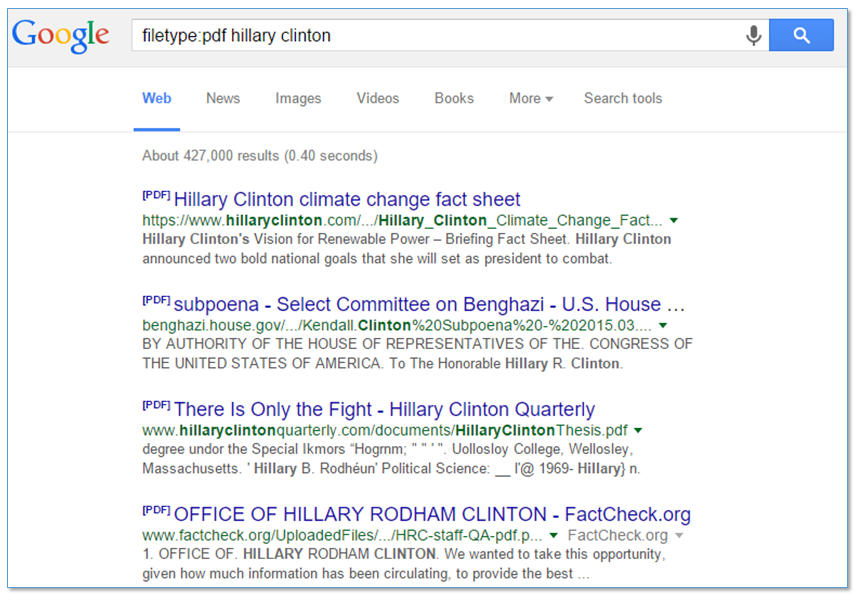The image depicts a Google search results page, which is wider than it is tall. Centered prominently within the image is a search results box with a thin blue border and a subtle drop shadow on the right side and bottom, creating a slight 3D effect. The background of the page is predominantly white, except for a light gray banner at the top.

In the upper left corner of the page, the recognizable Google logo is displayed. Directly beneath the banner, there is a search box containing the query: "filetype:PDF Hillary Clinton." This search specifies a search for PDF files related to Hillary Clinton, who is noted as a former Secretary of State, First Lady, and Presidential candidate. The search results indicate approximately 427,000 results, with the "Web" search option selected.

The top of the screen displays four highlighted PDF files:

1. **Hillary Clinton Climate Change Fact Sheet**
2. **Subpoena from the Select Committee on Benghazi, U.S. House** - accompanying commentary mentions the chaotic nature of this event.
3. **Only the Fight: Hillary Clinton Quarterly**
4. **Office of Hillary Rodham Clinton, FactCheck.org**

The caption reflects on the usefulness of using specific search operators, such as "filetype:PDF," to refine search results on Google, which can be particularly helpful for targeted research. The functionality allows the user to filter results to specific file types, offering greater precision in search outcomes. This search method is suggested as a valuable tool to remember for future internet research endeavors.